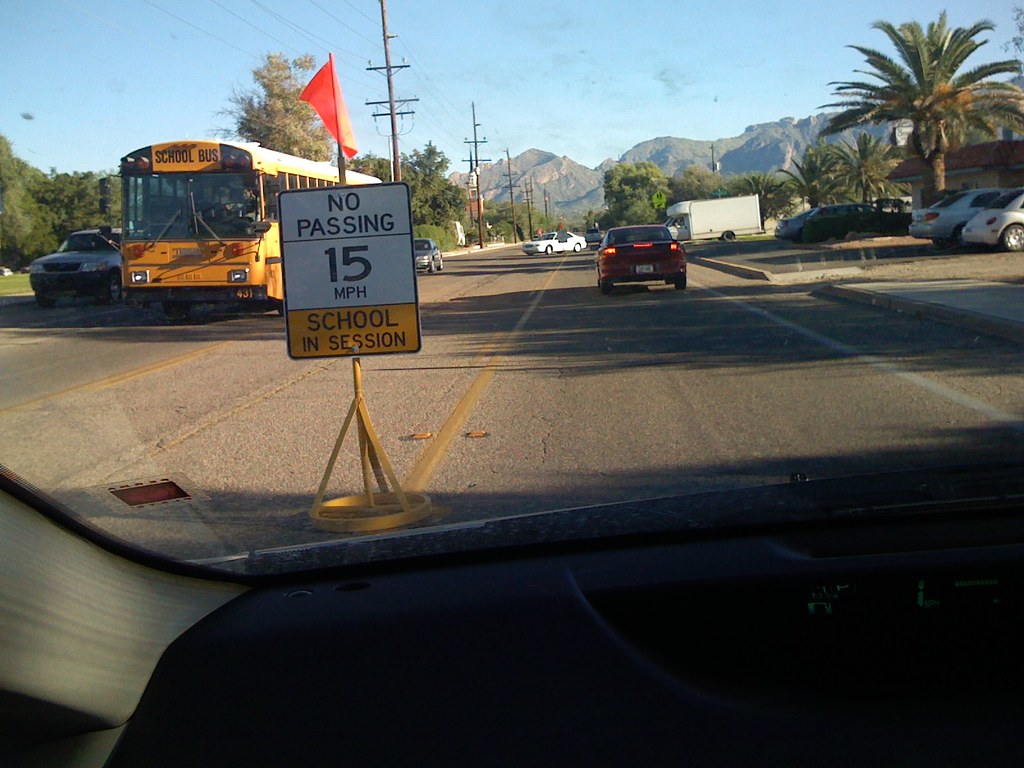The photograph captures a vibrant scene in a tropical locale, as evidenced by the tall palm tree prominently visible in the image's top-left corner. The perspective shows the view from within a car, although it’s unclear whether the shot originates from the front or rear seat due to the limited visibility of the dashboard. Through the windscreen, a bustling road unfolds, featuring a prominently displayed road sign indicating a "no-passing" zone and a speed limit of 15 miles per hour due to an active school session. A yellow school bus is positioned on the opposite side of the road, with another vehicle waiting behind it. A few cars are in the line ahead, while additional vehicles are parked off to the side in a lot. In the background, a striking range of jagged mountains stretches into the horizon, adding an element of rugged natural beauty to the tropical setting.